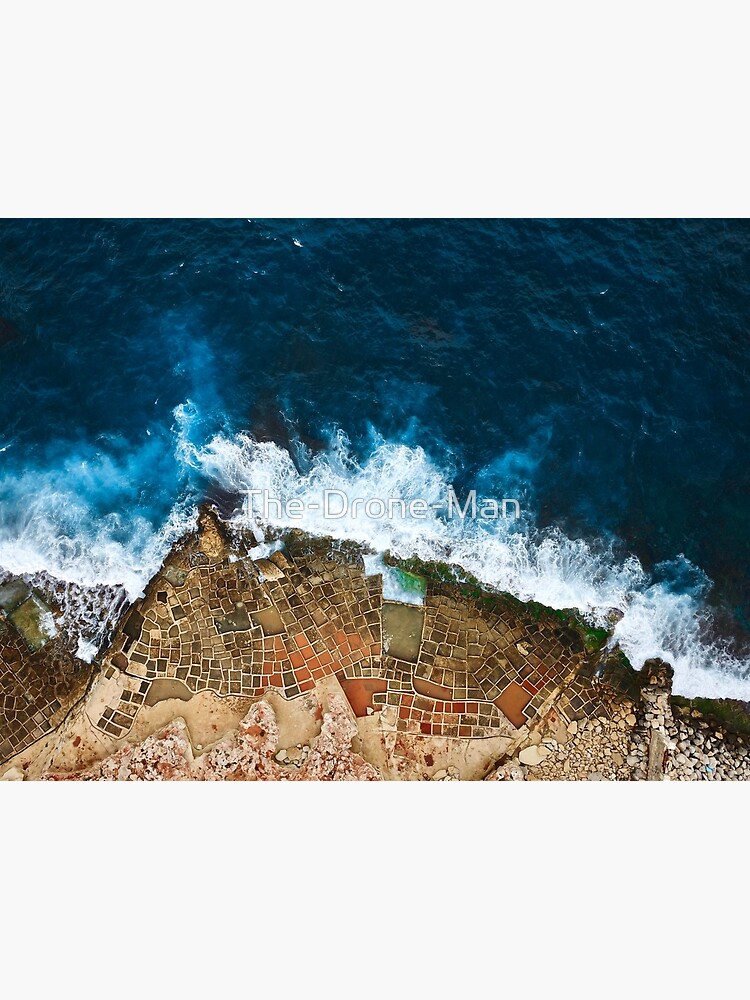This aerial photograph captures the mesmerizing interface between land and ocean, clearly divided with the ocean occupying the top half and the land the lower half of the image. The ocean, a deep and enchanting mix of dark turquoise and blue, is animated with ripples and crashing waves, which create a haze of white foam as they meet the shore. The land, characterized by a fascinating patchwork of various squares and rectangles, contrasts sharply with the dynamic water. These sections are delineated with clear boundaries and display an array of colors, including tan, reddish-orange, brown, and sand. Scattered amidst the land are numerous rocks of different sizes and shades, with larger gray stones nearer to the water. Adding complexity to the scene, a hint of green vegetation is visible at the shoreline. Central to the image is a conspicuous watermark that reads "the Drone Man." This stunning and intricately detailed aerial view effectively captures the vibrant interplay between the structured land and the ever-moving ocean.